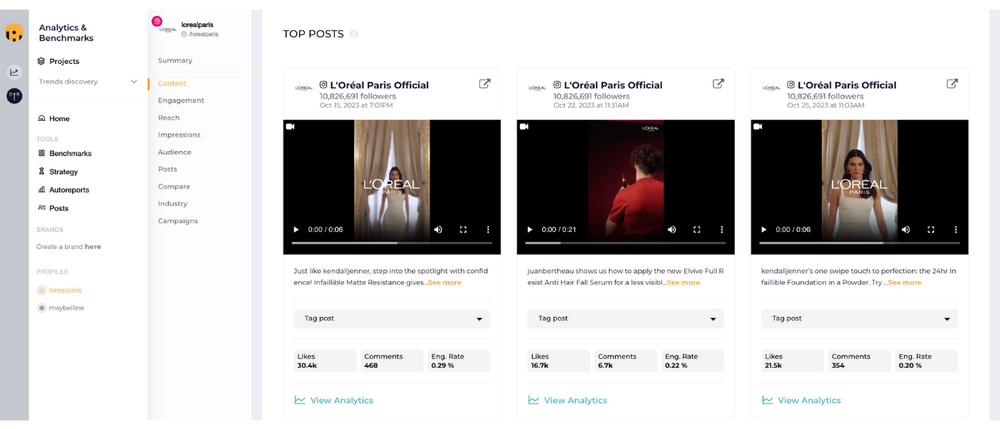A wide screenshot of a computer monitor displaying an analytics dashboard. The interface features a vertical gray strip on the left side with three circular icons in orange, gray, and black at the top. The main interface, slightly blurry and filled with text, is split into two columns. 

On the left side, the column is labeled with the header "Analytics and Benchmarks." Directly below in black is the label "Projects." This column's content includes bold, black headers reading Home, Benchmarks, Strategy, Auto Reports, and Post, each accompanied by a matching black icon.

The right side of the monitor showcases another column starting with a pinkish dot containing some white detail, though its exact purpose is unclear. This column has a blurry black label at the top with the legible word "Summary." Below that label, a series of black-text headings are listed, including Engagement, Reach, Impressions, Audience, Post, Compare, Industry, and Campaigns. An orange label selection stands out among these headings.

Additionally, there are three video thumbnails aligned vertically on this side, all under the heading "Top Post." Each thumbnail shows varying progress bars indicating different amounts of video played. The first video is titled "L'Oreal Paris Official," followed by its preview. Below are interactive elements including a dropdown menu labeled "Tag Post," and three sections labeled Likes, Comments, and ENG Rate (presumably for Engagement Rate). At the bottom left of each video preview is a bar chart icon next to the label "View Analytics."

Both the second and third video previews are similarly structured, with each section beneath the video marked with the same labels: "Tag Post," "Likes," "Comments," "ENG Rate," and "View Analytics." Each video is associated with the "L'Oreal Paris Official" account.